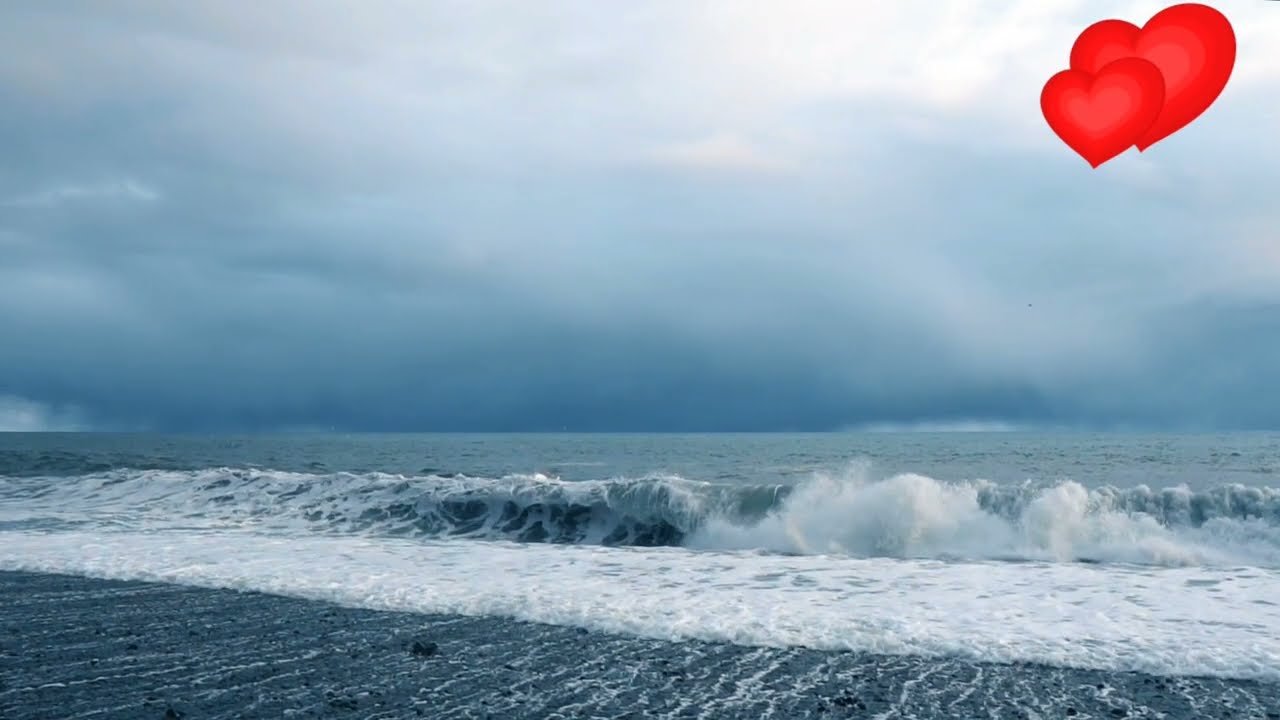This full-color photograph captures a dramatic beach scene taken from the shore, showcasing nature in its untamed beauty. The beach, composed of black sands scattered with rocks and pebbles, juxtaposes strikingly with the blue ocean. A sizable wave crashes near the shoreline, creating a foamy white froth. Further out, the water appears relatively calm. Above, the sky is densely packed with dark, foreboding clouds, suggesting an imminent storm. In the distance, it appears to be raining, though the immediate beach area remains dry. Visually distinct in the top-right corner are two digitally added red hearts, with a smaller heart superimposed onto a larger one, adding a touch of juxtaposed warmth to the otherwise moody scene.